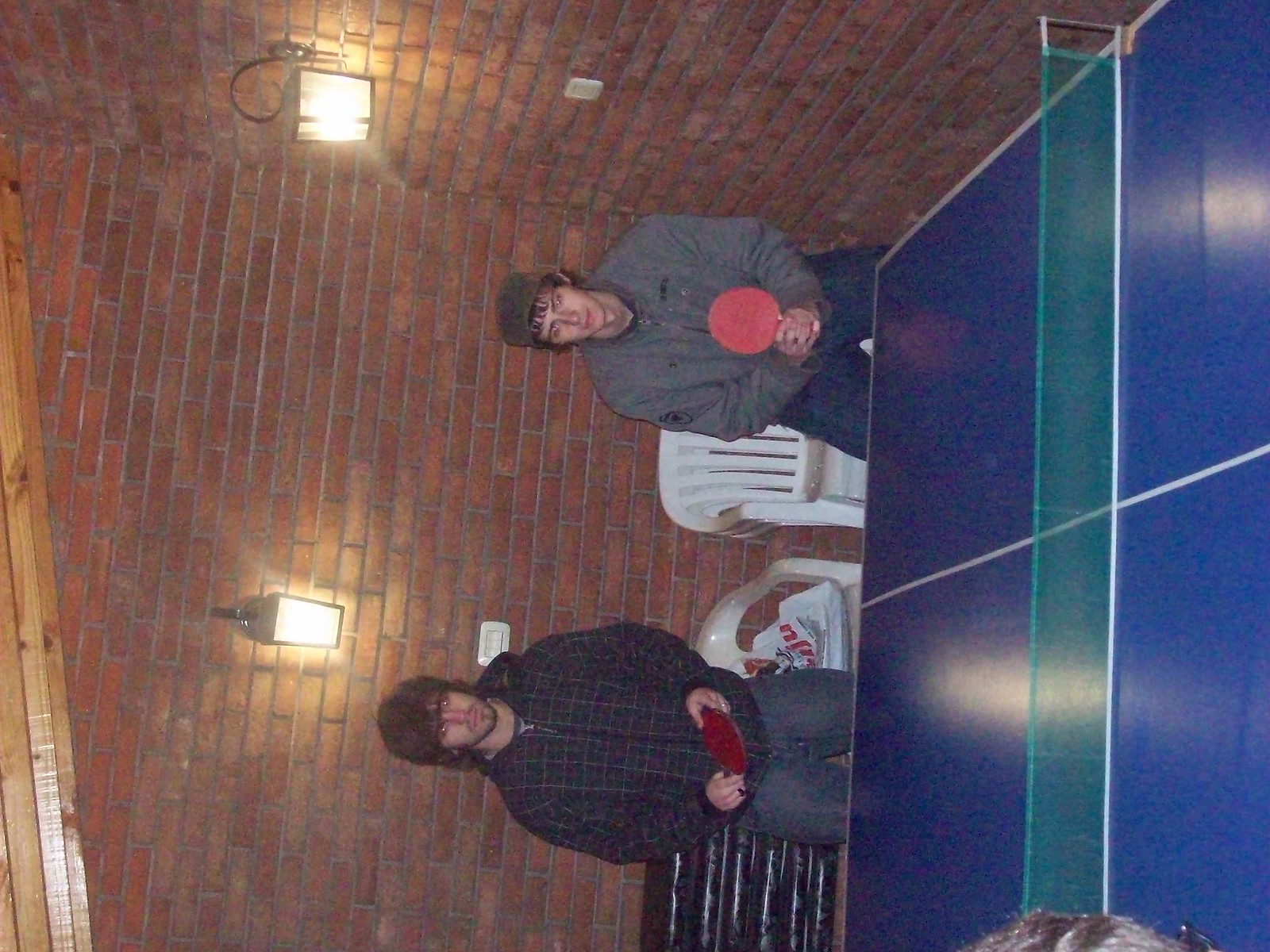The photo captures an indoor scene featuring two men standing side by side at one end of a blue ping-pong table, which has a green net. Both men, who appear to be playing as partners, hold red ping-pong paddles. They are positioned in front of a red brick wall, where two white plastic chairs are visible. Above each man, a lit lantern is attached to the wall. The man on the left, who has long shoulder-length brown hair, is wearing a dark hoodie and jeans. The man on the right, with shorter brown hair under a gray beanie, is dressed in a gray jacket and blue jeans. The lighting and simple background emphasize the players and their game.